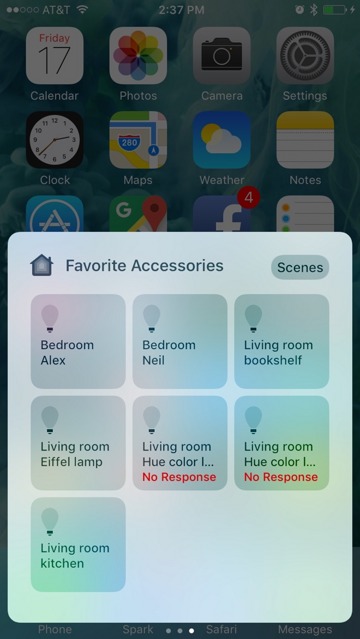This image is a screenshot of a smartphone displaying various details and icons. At the top, the status bar shows the AT&T carrier name with a signal strength indicator displaying two out of five filled dots. Additionally, there is a Wi-Fi symbol, the time marked as 2:37 PM, an alarm clock icon, a Bluetooth symbol, and a battery that is half full.

The screen is filled with app icons, with a white interface box occupying a little over half of the bottom portion. This box includes an illustration of a house frame and the header "Favorite Accessories and Scenes." Below that header are seven square icons arranged in a grid: three across the top row, three across the middle, and one on the bottom row. The items listed are:
- Bedroom Alex
- Bedroom Neil
- Living Room Bookshelf
- Living Room Eiffel Lamp
- Living Room Hue Color (appearing twice)
- Living Room Kitchen

Each square has a light bulb icon, suggesting control over various lighting or smart home accessories.

In the background, app icons include Calendar (showing "Friday the 17th"), Photos, Camera, Settings, Clock, Maps, Weather, Notes, Facebook, and Google Maps.